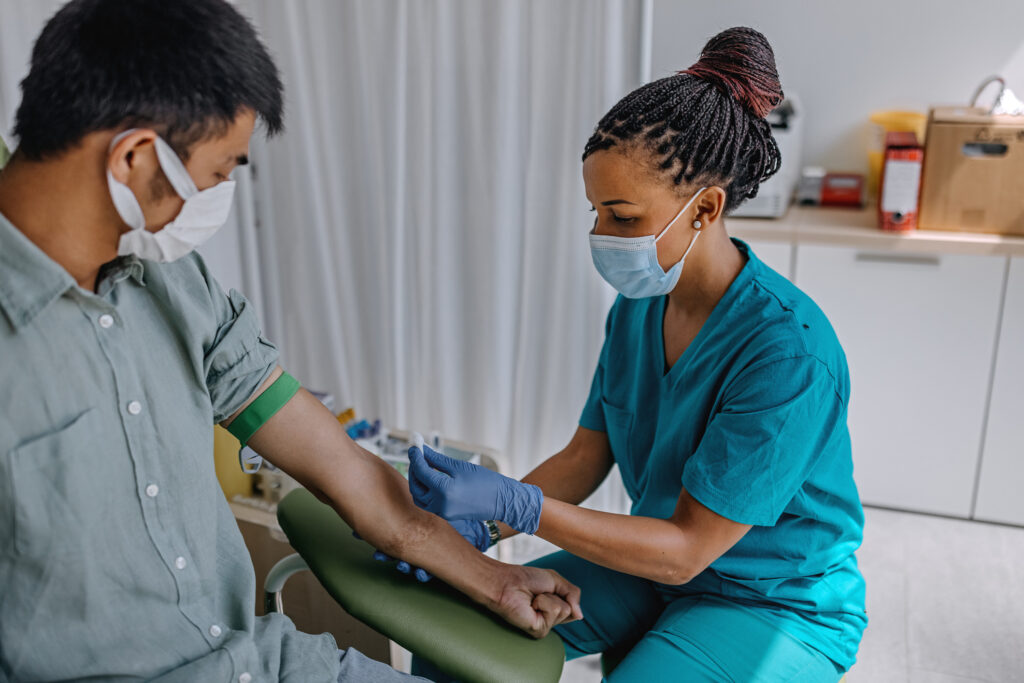In a high-quality photograph taken in a medical office, an African American nurse is seen preparing to draw blood from a patient. The nurse, appearing to be in her early thirties, is dressed in dark green medical scrubs and is wearing blue latex gloves. Her face is partially covered by a blue mask secured with straps behind her ears, and her long, braided hair is neatly pulled back into a bun. She is seated on a stool to the right of the image, holding a cotton swab as she swabs the man’s arm.

The patient, a young man with black hair, is sitting in a specially designed chair on the left side of the image. His arm rests on a large green cushion, and a green band is tied around his bicep, suggesting he's about to have his blood drawn. He, too, is wearing a mask – a white cloth one with straps behind his ears. The man, with a brown complexion, is dressed in a button-up shirt, which may be either light gray or blue, and has his sleeve rolled up to facilitate the procedure. 

The background consists of a long white curtain and shelves holding various items, complementing the clinical setting of the room. The detailed composition captures a moment of medical care, highlighting the precautions observed possibly during the COVID-19 pandemic.